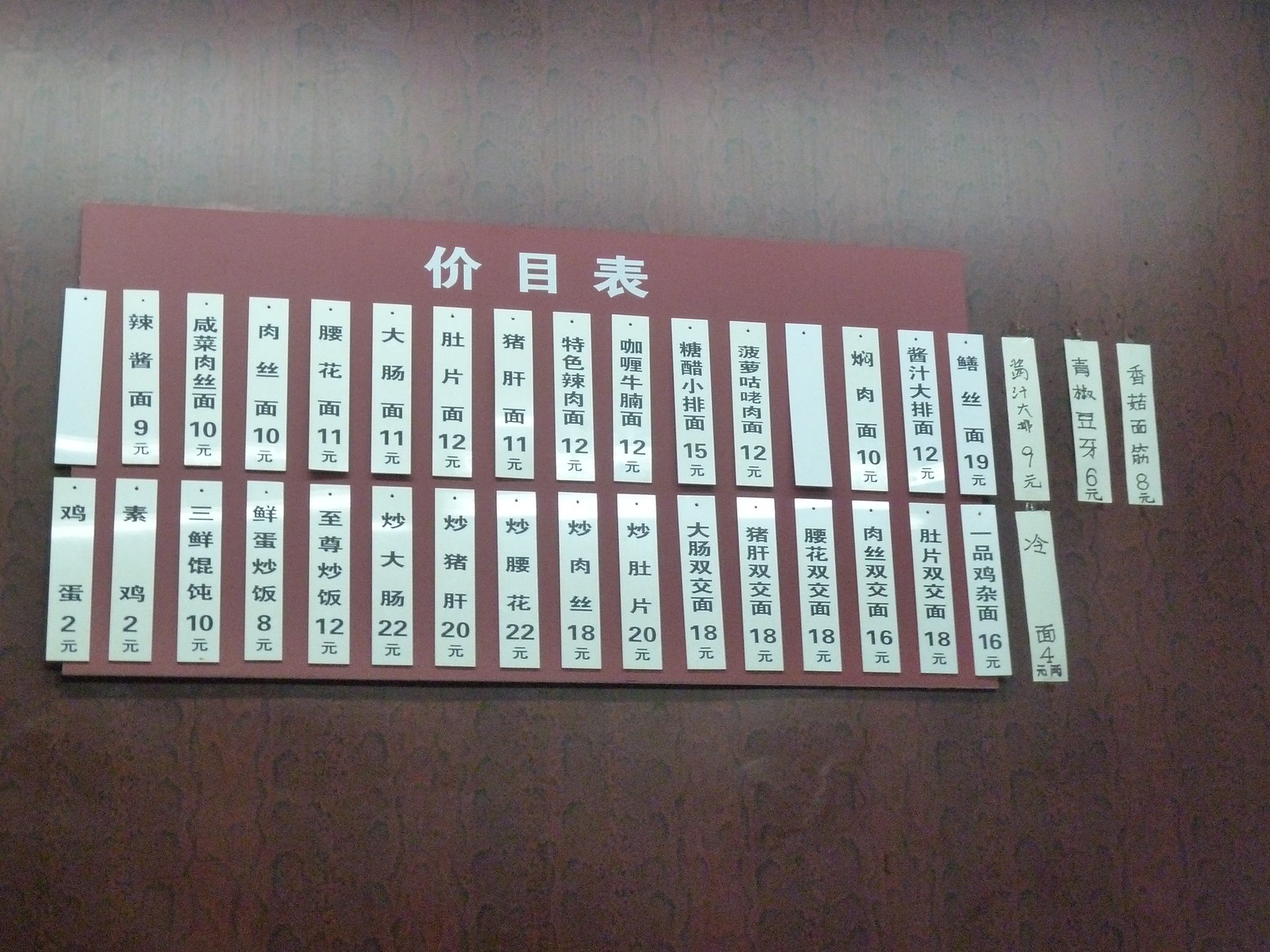A vibrant color photograph showcases a scene rich with cultural elements. At the forefront, a robust brown wooden table serves as the foundation. Resting atop is a striking red board adorned with several white strips of paper or ribbons, each meticulously placed in a vertical arrangement. The delicate papers bear inscriptions in an Asian script, creating an enigmatic yet visually appealing pattern that flows from top to bottom.

Towards the bottom edge of each strip, numerical characters are prominently displayed: 9, 10, 10, 11, 11, 12, 11, 12, 12, 15, 12, 10, 12, 19, 2, 2, 10, 8, 12, 22, 20, 22, 18, 20, 18, 18, 18, 16, 18, and 16. These numbers add a layer of intrigue, suggesting some form of ranking or categorization within the context of the writing.

Additionally, several other paper strips stand alone, positioned off to the side, somewhat detached from the main assembly. This thoughtful composition is visually enriched by the contrast between the warm brown wood and the vibrant red backdrop, accentuated by the crisp white of the paper strips, offering a visually engaging and culturally rich tableau.